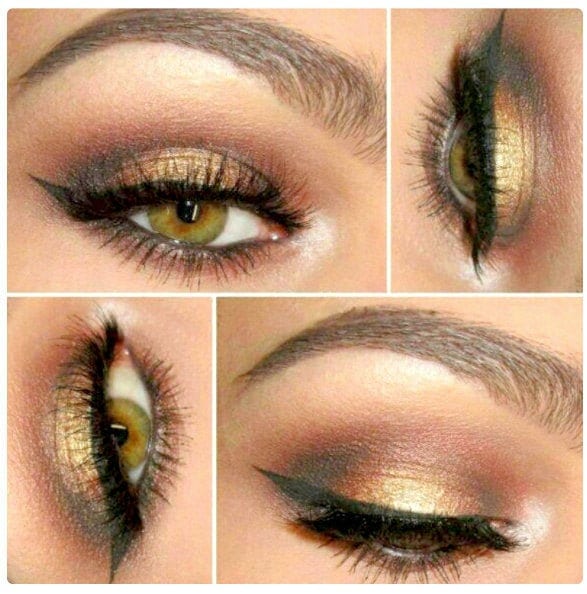The image is a square grid composed of four close-up photographs of a striking light green human eye with well-groomed eyebrows, adorned with mascara and gold eyeliner. The upper-left rectangle features the eye in its natural orientation, wide open, showcasing the detailed makeup. Adjacent to it, the upper-right rectangle presents the same eye rotated 90 degrees clockwise, maintaining the vivid makeup details. Below it, the lower-right rectangle displays the eye semi-closed, turned another 90 degrees clockwise, exhibiting the eyeliner on the closed eyelid prominently. Finally, the lower-left rectangle mirrors the upper-left image but tilted 90 degrees counterclockwise. Together, these images intricately portray the eye from various angles, highlighting the meticulous makeup artistry.